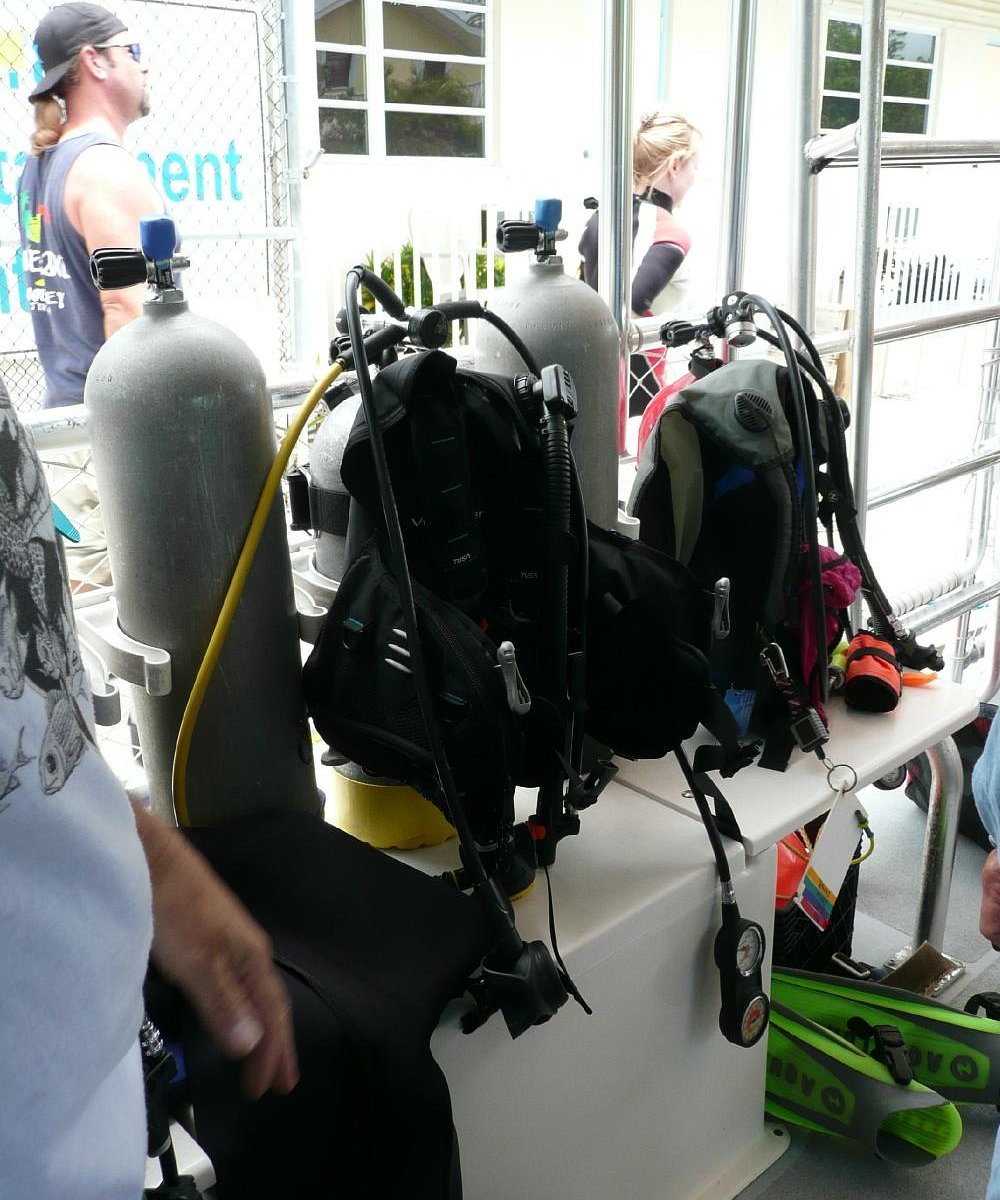The image depicts a taller-than-wide, rectangular color photo of a scuba shop or scuba gear rental setup. Central to the image, there is a white table holding scuba diving equipment, prominently featuring two tall, thick gray tanks with black and blue nozzles on top. The tanks appear to be oxygen tanks, and attached to them are black backpacks with various attachments. Among these attachments are black tubes and a distinctive yellow tube, which suggests they may be part of a breathing apparatus. On the left side of the table, some neon green elements are visible, possibly additional scuba gear components.

In the foreground at the bottom left, there's a partial view of a man's left arm, who is wearing a light blue shirt with a black design, though the image of his arm is somewhat blurry. Additionally, part of a woman's chest dressed in scuba attire is seen in the same corner.

The background reveals more context: on the top left, there is a man wearing a backwards cap, a blue tank top, and sunglasses, suggesting a casual outdoor setting. To the right of him, closer to the center background, stands a blonde woman, apparently also in scuba gear. These individuals are positioned in front of a white building with windows and some metal poles visible along the area. Outside the building, a chain link fence gate can be seen, reinforcing the appearance of an organized scuba rental facility.